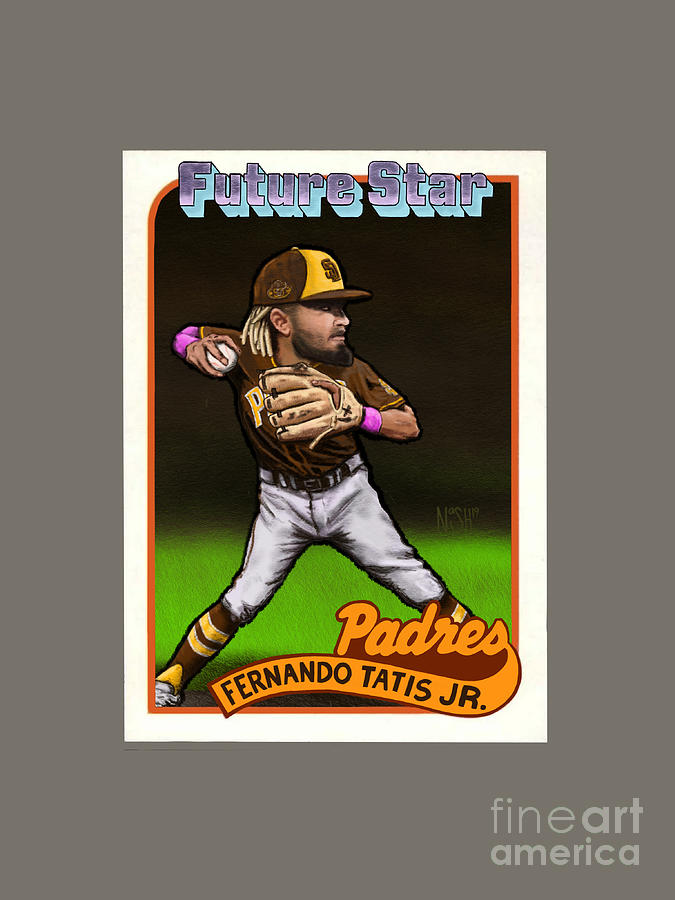This detailed image features a simulated baseball card of Fernando Tatis Jr., a player for the San Diego Padres. The card, which has been digitally modified, involves a play on the Padres team with the name 'Fernando Tatis Jr.' clearly displayed. The card depicts an animated character, dressed in a San Diego Padres uniform and cap, pitching a ball. At the top, the card prominently reads "Future Star" in purple text against a blue background. Fernando is looking towards the right side of the image, wearing purple wristbands. The card, which has a white border and sits on a gray background, is marked with "Fine Art America" on the lower right part. The overall background of the image is predominantly gray.